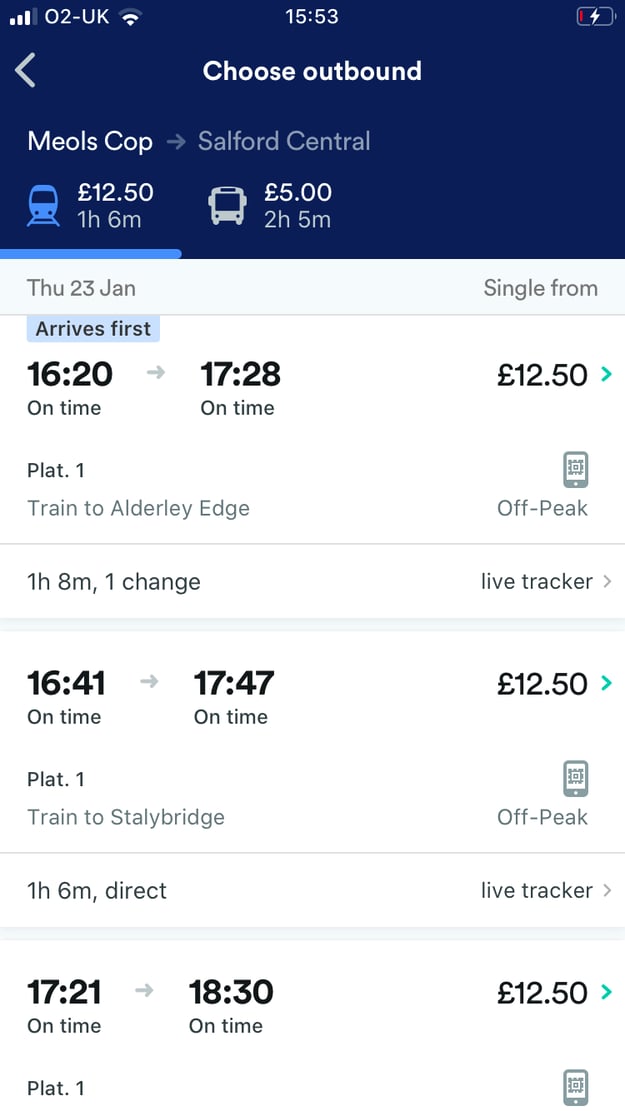In this detailed screenshot from a tablet or cellular device, the time displayed at the top is 15:53. On the right side of the status bar, a low battery icon with a charging symbol can be seen, indicating that the device is currently charging but has a low battery level. To the left, there are wireless signal indicators. The interface has a primarily white theme accented with a blue top banner, along with sections of black and gray text. 

At the top of the screen, the blue banner contains the text "Choose Outbound" in white. To the left of this text, there is an arrow pointing left. Directly below the banner, the screen displays travel options starting with a header "Meals Cop to Salford Central." This includes a train icon followed by the fare "$12.50," a duration of "One hour and six minutes," and another travel option with a bus icon, indicating a fare of "$5" and a travel duration of "Two hours and five minutes."

Further down, detailed travel schedules are listed. The first section starts with the arrival time of "1620 to 1728" and mentions "On Time" twice, indicating punctual service. The journey is described as a "Platinum One Train to Alderley Edge," lasting "One hour and eight minutes" with "one change." The fare for this off-peak option is listed as "$12.50," and the section also mentions a "live tracker." The date provided is Thursday, 23rd January.

Overall, the screenshot methodically displays different travel options, times, prices, and other relevant details for journeys from Meals Cop to Salford Central, providing a comprehensive overview for potential passengers.